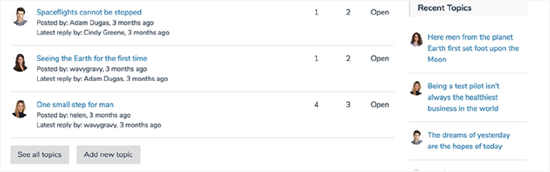In this slightly blurry screenshot set against a white background, multiple discussion posts are visible. 

In the top left corner, there is an image of a man with brown hair. To the right of his face, the text in blue reads, "Space flights cannot be stopped." This post was made by Adam Dugas three months ago, with the latest reply by Cindy Green also posted three months ago.

Beneath this post, there is the next discussion, with the blue text reading, "Seeing the Earth for the first time." The accompanying user image shows a female with dark hair. This post was made by Wavy Gravy three months ago, and the latest reply was by Adam Dugas three months ago.

Following that, another user post is visible featuring a female with long blonde hair. The blue text for this post reads, "One small step for man," followed by black text indicating it was posted by Helen three months ago.

At the bottom of the screenshot, there are two gray buttons. The first button reads, "See all topics," and the second button reads, "Add new topic."